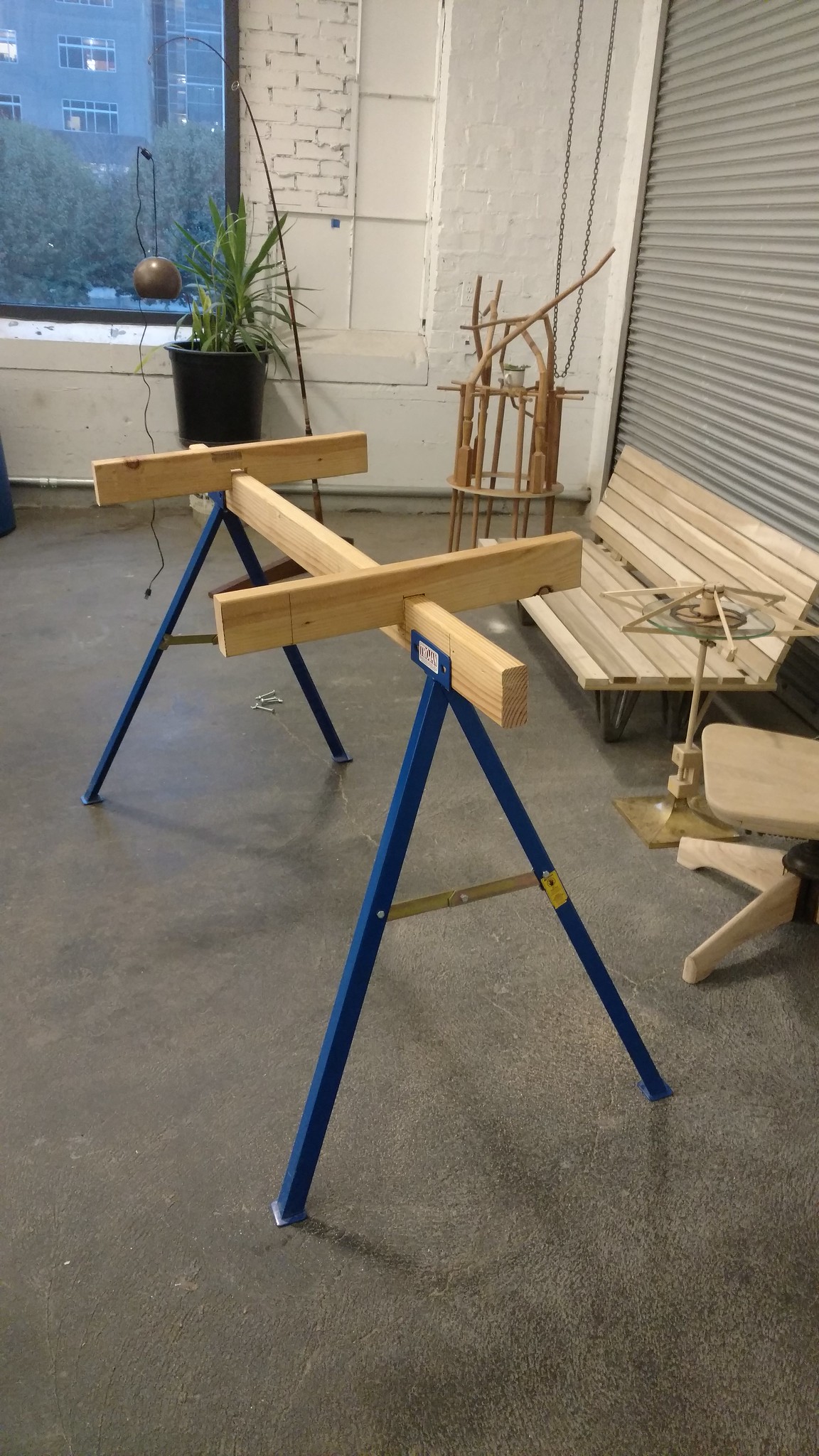This tall, narrow photograph captures a detailed interior scene set within what appears to be a woodworking shop. The focal point of the image is a sawhorse constructed from blue metal legs forming an upside-down 'V' shape, with a gold bracket running through the center for stability. Resting atop the sawhorse is a long 2x4 piece of wood positioned vertically, its front face oriented towards the right side of the image. Atop this main 2x4 are two shorter 2x4 pieces laid horizontally, each having a section cut out to fit snugly over the larger piece.

Surrounding this central setup are various woodworking elements and furniture. On the mid-right side, there are several pieces of wood and a wooden bench assembled from planks. Further to the right, a sculpted wooden chair and another wooden sculpture shaped with intricate, antler-like forms capture the viewer's attention. A black pot with a lush plant and a lamp contribute to the workshop's eclectic vibe.

In the background, a shut garage door leads to a white concrete brick wall. The wall features a large window through which the late evening light filters, revealing trees and the silhouettes of large buildings outside. The scene as a whole portrays a well-utilized creative space with a mix of functional and decorative woodworking.